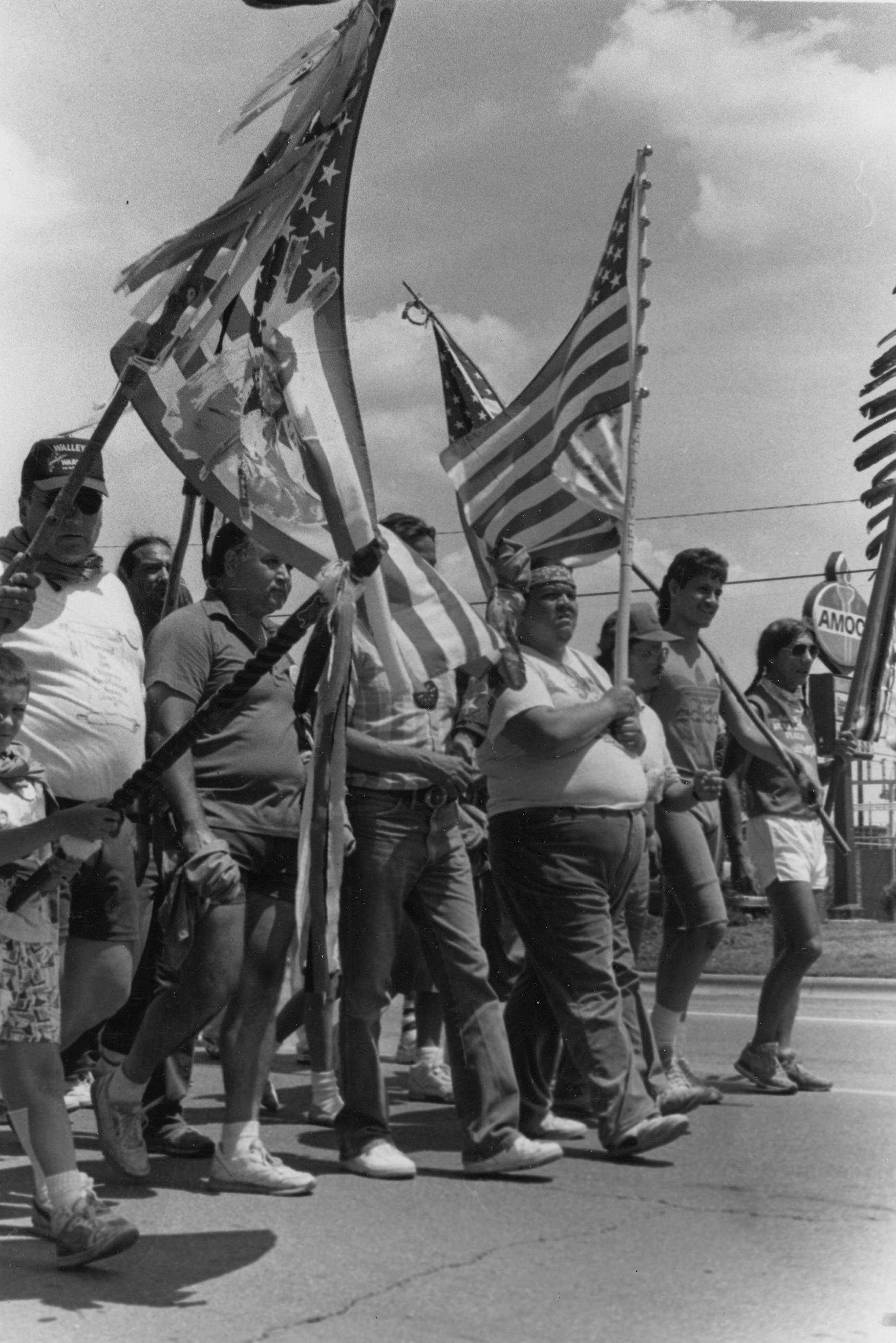The black-and-white photograph captures a diverse crowd marching down an asphalt street, holding American flags and another flag with Native American motifs, complete with cloth drapings hanging from the poles. The participants, who appear to be of Native American descent, don a mix of shorts, long denim pants, and traditional head adornments, including braided hair and thematic headbands. Men, women, and individuals of various ages are visible in the march. The event seems to be set in a modern time, although the monochrome filter adds a historical feel. The backdrop includes a partially obscured AMOCO gas station sign on the right side, suggesting the photo may hail from an era such as the 1960s. The sky above is cloudy, indicating overcast weather during the daytime.